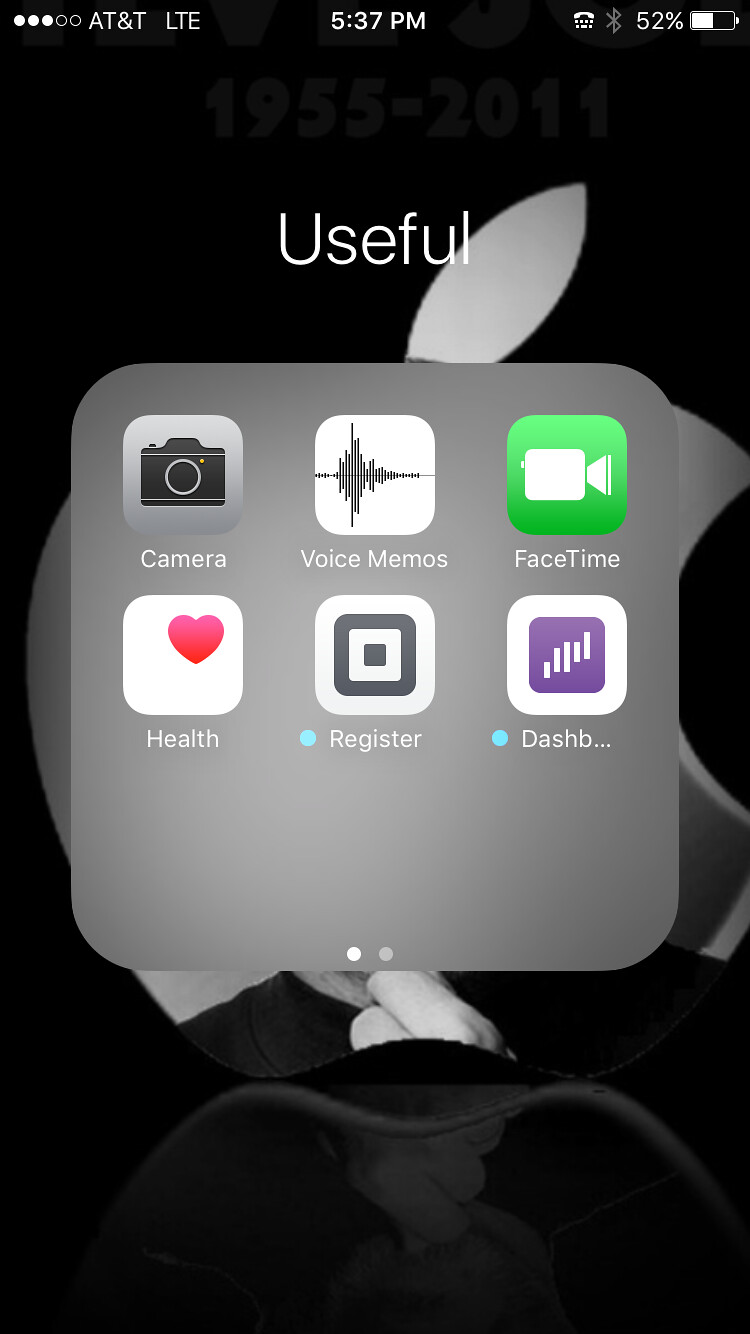In this detailed screenshot of an Apple iPhone, the screen displays various elements that give us insight into the device’s current status and user activity. At the top of the screen, the service indicator shows three out of five circles filled, indicating moderate signal strength. The carrier is AT&T, and the device is connected to LTE Wi-Fi. The time displayed on the iPhone is 5:37 PM, and the battery is at 52% charge.

The image showcases a folder titled "Useful" that is open, revealing its contents. This folder contains two pages of apps, although only the first page is visible in the screenshot. The visible apps include Camera, Voice Memos, FaceTime, Health, Register, and another app partially obstructed but identifiable as likely being Dashlane, indicated by the visible letters "D-A-S-H-B." Notably, the Register and Dashlane apps have a small blue dot next to their icons, signifying that they have been newly updated or recently installed.

The iPhone’s wallpaper prominently features the Apple logo, which incorporates a partial image of a person. The visible portion of this image shows the top of someone's shoulders and a hand, but much of the background is obscured by the app icons on the home screen. This detailed configuration hints at both the personalization and practical app organization preferences of the iPhone user.